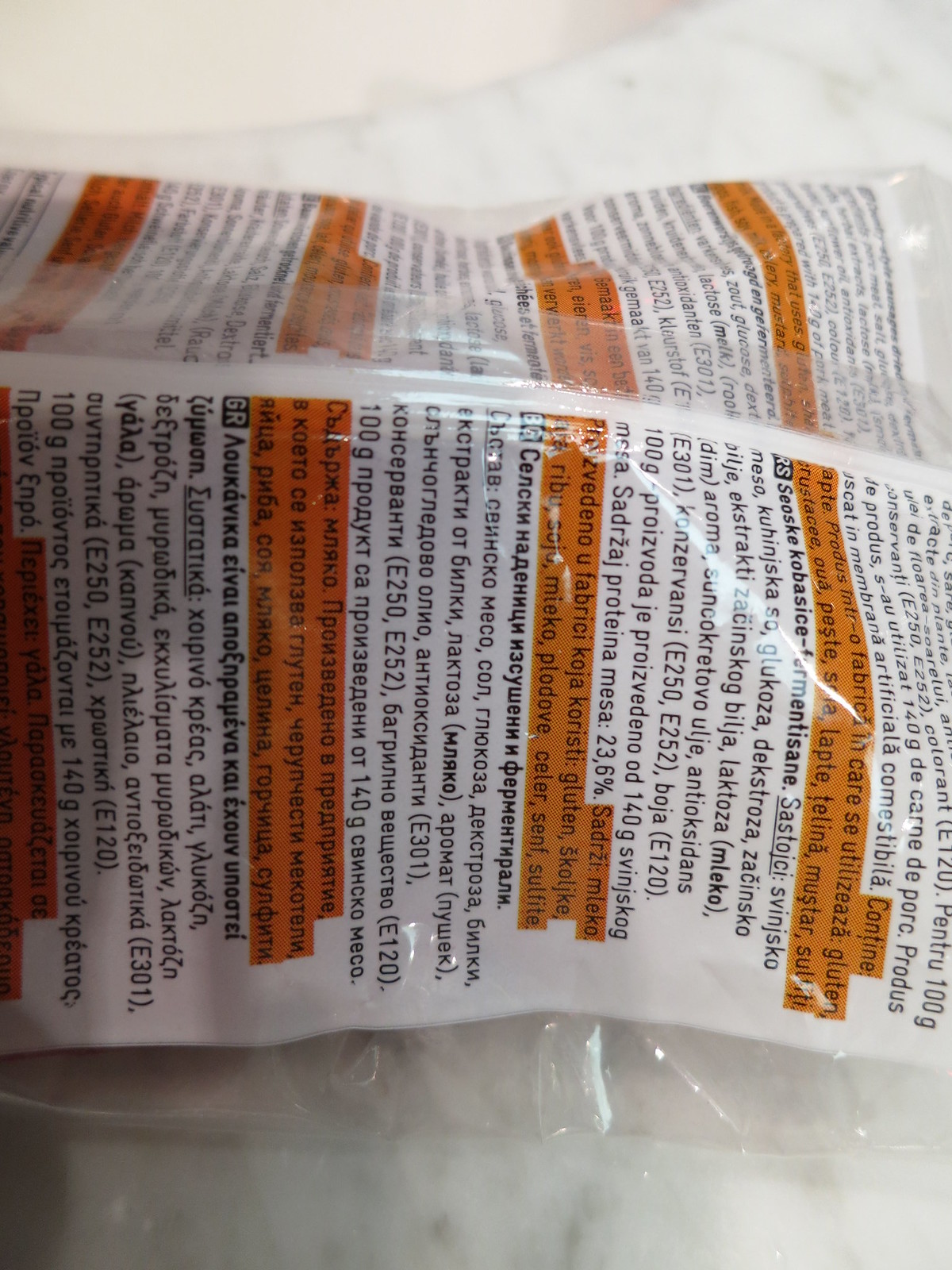This is a high-resolution photograph capturing a plastic package resting on a white surface. The package is predominantly orange with a white strip running down its center. It features text in a foreign language, printed in black font. The glossy surface of the plastic packaging reflects light, creating subtle highlights, while soft shadows cast at the bottom add depth to the image. The pristine white surface underneath also shows faint reflections of the lighting, contributing to the photograph's overall clarity. This focused composition emphasizes the package and its distinctive colors and textures.